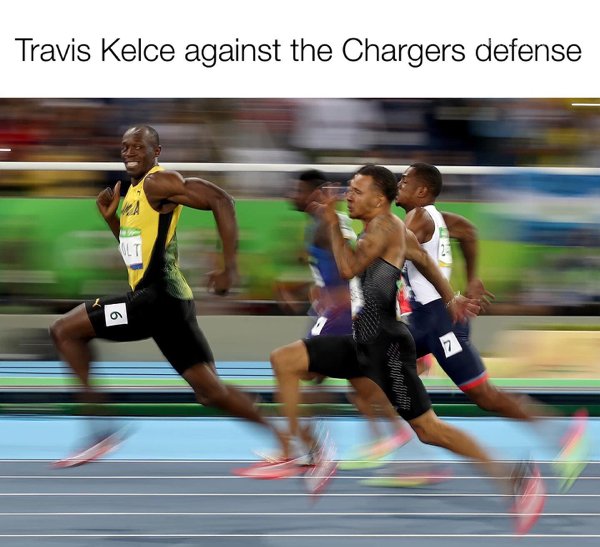In the image, a meme depicts Usain Bolt leading a race with a confident smile and giving a thumbs-up while three other runners struggle to keep up behind him. Bolt is dressed in a yellow and black athletic outfit with a number six on his black shorts and "Puma" written in white. His yellow top features barely discernible black text and the letters "LT" on a backdrop of green and blue. The track is marked with thin yellow lines, and behind the runners, a gray wall with blue and green stripes adds some detail to the blurred background. The other runners include one in blue, one in black, and one in a white shirt with blue and red-trimmed shorts. Above the image, a caption humorously reads, "Travis Kelsey against the Chargers defense," referencing the notable disparity in performance between Bolt and his competitors.